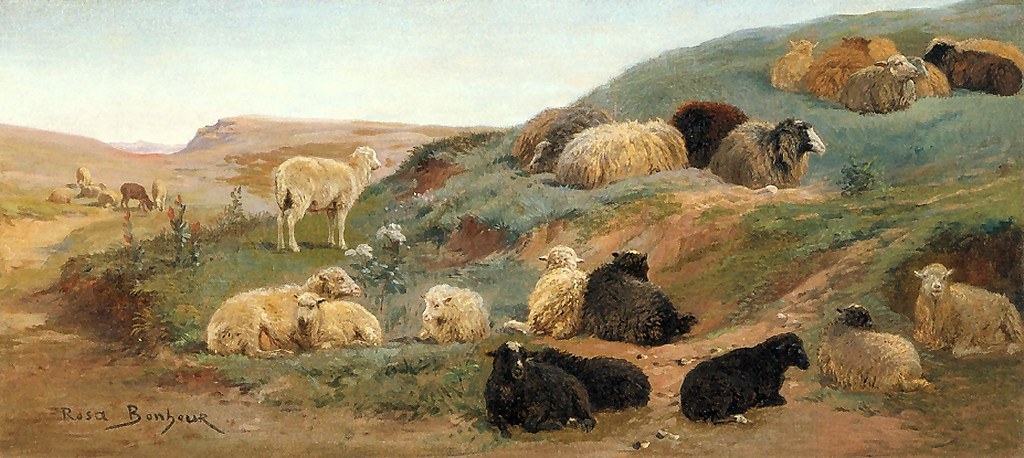In this detailed painting by Roscoe Bonheur, the scene depicts a tranquil desert landscape with a backdrop of a vibrant blue sky scattered with wispy clouds and a distant mountain range. The foreground is dominated by earthy brown dirt and rocks, transitioning into a lush, green grassy hill to the right. At the base and crest of this hill, a mixed flock of sheep recline and graze. There are approximately five to six white sheep, four to five black sheep, and several brown and tan ones. Among them, a single white lamb stands alert while others lie peacefully. A trio of black sheep is prominently placed in the middle foreground, contrasting beautifully with the green meadow. Scattered across the hill, the sheep are arranged in small clusters, indicating a variety of positions and activities, with some grazing quietly. Off in the distance, smaller indistinct figures suggest more animals, possibly sheep or even horses, adding depth to the painting. The serene composition is intricately signed "Roscoe Bonheur" in black lettering at the left-hand corner, affirming the artist's ownership and enhancing the authenticity of this picturesque scene.